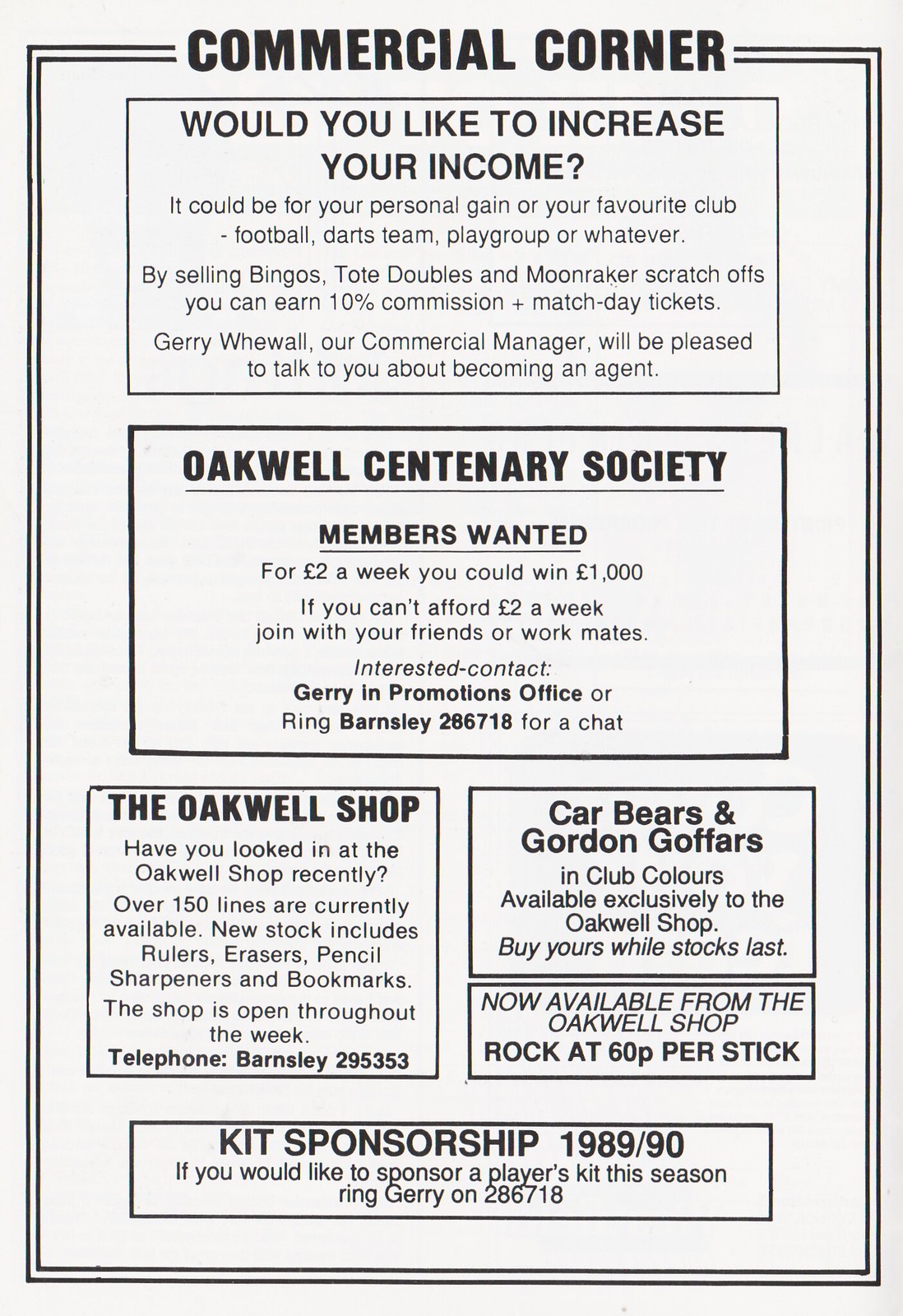This image is a vintage advertisement with a double black border on a white background, prominently titled "Commercial Corner." The top section features the headline, "Would you like to increase your income?" and outlines several opportunities, such as selling bingos, tote doubles, and Moonraker scratch-offs, with the incentive of earning a 10% commission and match-day tickets. Jerry Wehwalt, the commercial manager, is introduced as the contact person for those interested in becoming an agent, available in the promotional office or via phone at Farsley 286718.

Below this, a bolded section highlights an invitation to join the Oakwell Centenary Society, targeting individuals with a weekly contribution of $2 and a chance to win $1,000. The ad encourages pooling resources with friends or coworkers if affordability is an issue.

Further down, the ad showcases two smaller sections promoting the Oakwell Shop on the left, and, on the right, it features ads for "Car Bears" and "Golden Gophers," with an additional note about rock candy priced at 60p per stick. The bottommost section invites sponsorship for player kits for the 1989-90 season, directing interested parties to contact Jerry at the same phone number. The advertisement is packed with various money-making and promotional opportunities, all coordinated through Jerry Wehwalt.